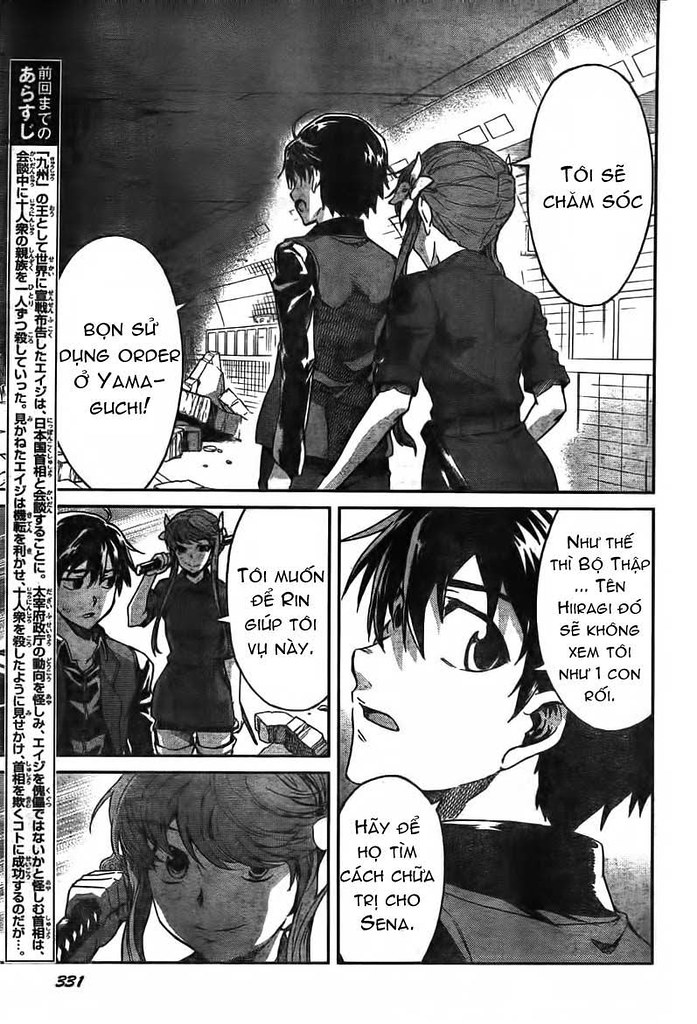This detailed black-and-white comic book page, reminiscent of anime or graphic novel art, features multiple frames filled with expressive characters and Japanese dialogue balloons. At the top of the page, set in what looks like an old, abandoned tunnel, a man with dark hair in a long jacket and a woman with long hair tied on both sides, dressed in plain black sleeves, are walking away from us. The man is speaking, but the dialogue is in Japanese, written inside white speech bubbles.

Below this, on the left-hand side, the first frame captures a girl in a knee-length dress aiming a flashlight at a boy who appears downtrodden, his head slightly bowed. The girl’s boots are just visible, and she is speaking to him, her words rendered in Japanese text balloons. 

In the adjacent frame below this, a close-up of a different person holding a sword in their right hand faces the viewer directly, their long hair cascading around their face as they assume an intense stance. Additional Japanese text accompanies this figure.

The final image on the right captures a dark-haired boy, possibly the same as described earlier, turning around mid-speech, and more Japanese text bubbles hover near his head.

Running along the left side of the page are rows of Japanese characters, possibly providing additional narrative context or dialogue from the characters. A small page number, 331, is visible at the bottom left corner, situating this scene within the broader story.